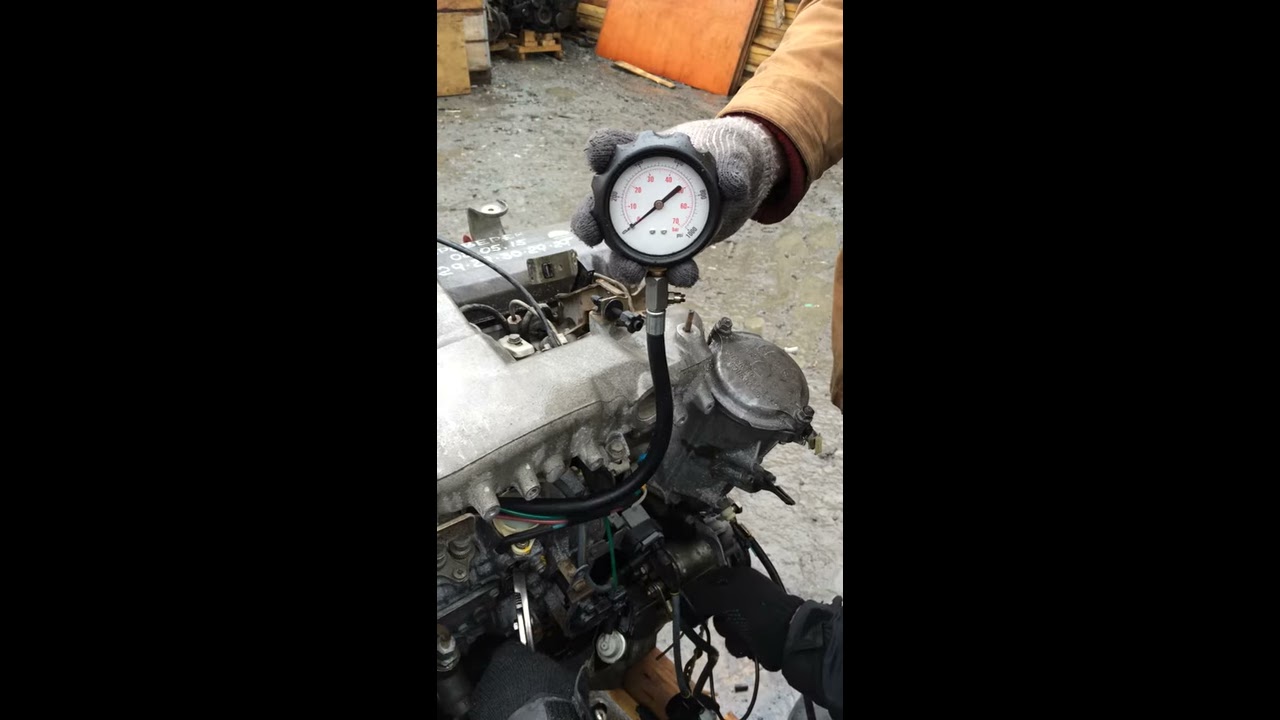This photograph, taken in portrait orientation, captures a detailed scene where two individuals are working on an exposed engine or machine in a workshop setting. The central focus of the image is the engine, which reveals various visible parts and tubes. One person, clad in black gloves and a black jacket, is actively working on the machine. Another hand, wearing a gray glove and a brown jacket, is holding an air compressor valve or meter, possibly to monitor the engine's performance metrics. The background consists of a rocky dirt floor with puddles of water and scattered wooden blocks and plywood, indicating a makeshift or temporary working area. Two vertical black strips frame the left and right sides of the image, adding to the industrial ambiance of the setting. The overall impression is of meticulous work being done to ensure the machine operates efficiently and safely.